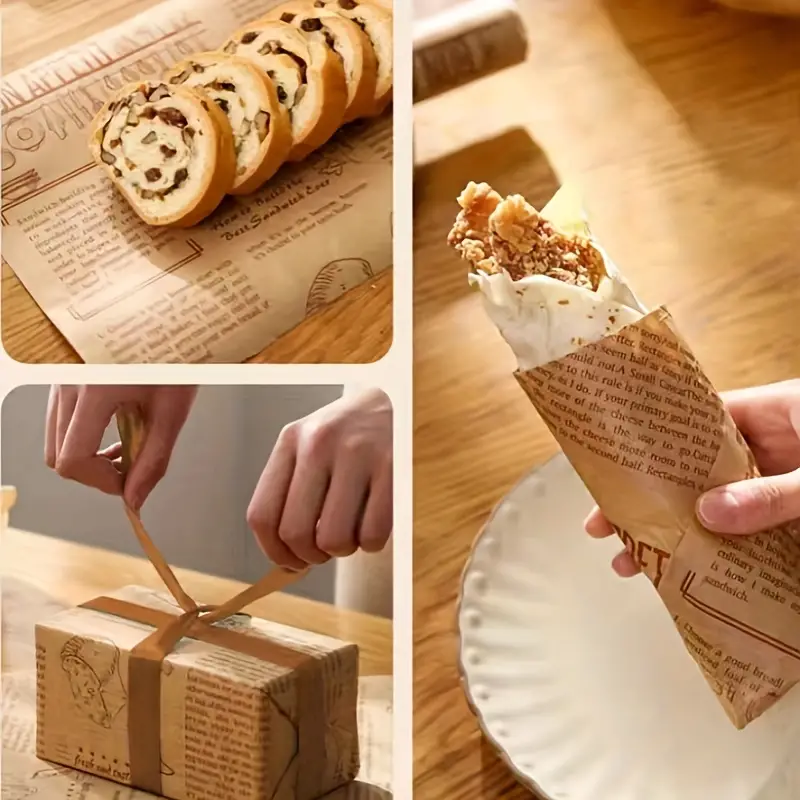This collage image is divided vertically, with two square photographs on the left and one long rectangular photograph on the right. Each image features a wood table background. 

In the top-left square image, slices of a nutty, possibly raisin-filled, loaf of bread are artfully arranged on a piece of brown wrapping paper inscribed with undecipherable text, suggesting a cooking theme. Directly below, the bottom-left square photograph captures a gift box wrapped in the same distinctive brown paper. Two hands are caught in the act of tying or untying a brown ribbon around the box, emphasizing a sense of anticipation or gift-giving. 

The right-hand side of the collage is dominated by a vertical photograph of a hand holding a tortilla wrap, filled with pieces of fried chicken. The tortilla is enclosed in a similar brown wrapping paper, printed with dark text, matching the cohesive design elements seen in the other images. Behind the wrap, a white plate is partially visible. 

Altogether, the images collectively evoke themes of homemade culinary delight and thoughtful presentation, unified by the consistent use of brown, text-patterned wrapping paper.